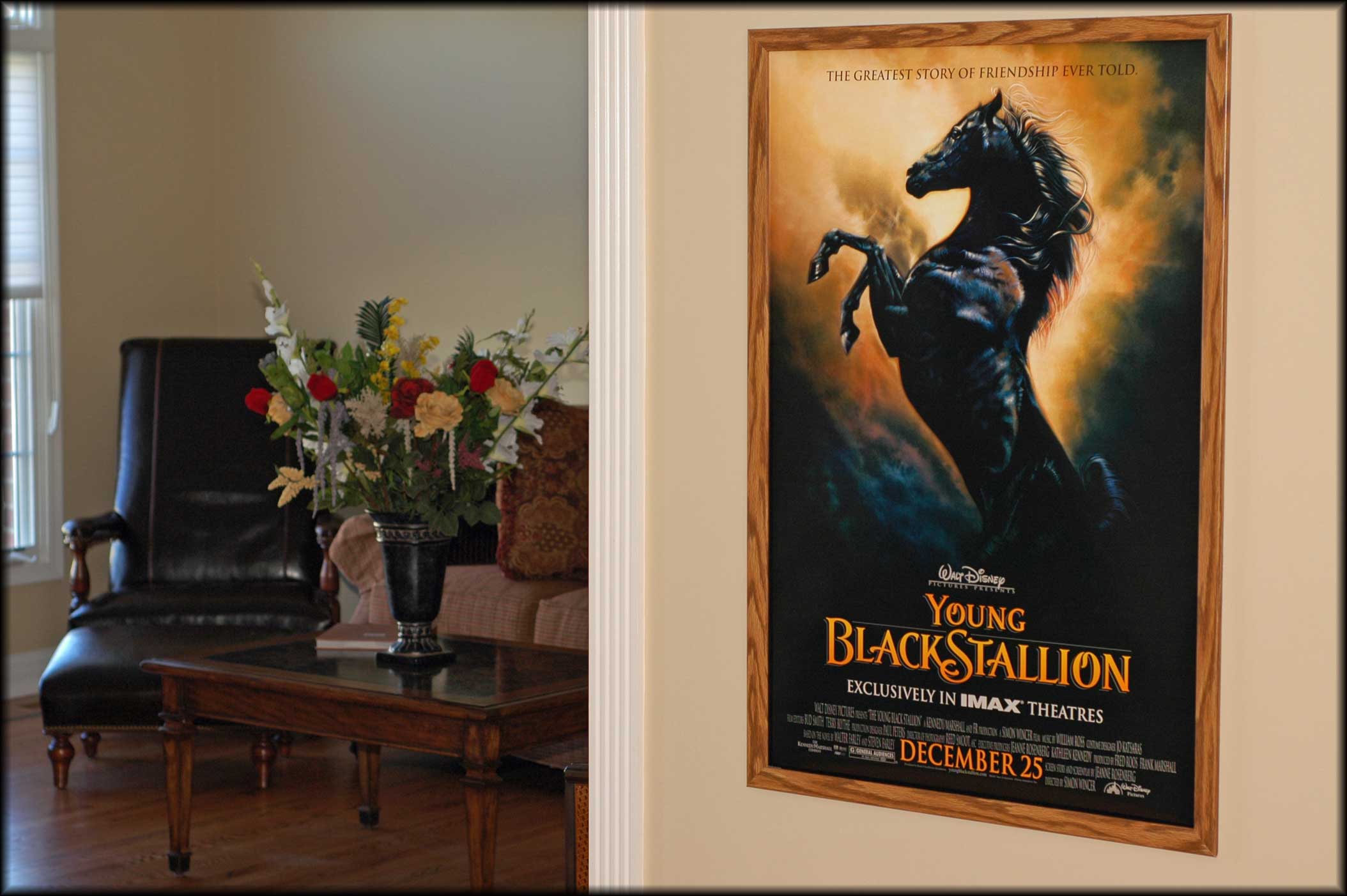This image captures a cozy interior of a room with cream-colored walls and wooden flooring. A large window occupies the left side, adorned with a sheer, white, curved curtain that reveals a glimpse of a balcony railing outside. The room is tastefully furnished, featuring a black upholstered sofa or chair, and a second sofa accented with pink and brown patterned cushions. A wooden center table with a glass top sits in front, adorned with a diary or book and a black vase brimming with colorful flowers.

Dominating the right wall, which is bordered in white, is a striking movie poster of "The Black Stallion" from the early 80s. The poster, illuminated and framed in wood, showcases a powerful black horse rearing on its hind legs against a fiery, yellow-orange backdrop. At the top, the impactful tagline "The Greatest Story of Friendship Ever Told" is written in black. Below, in white, it states "Walt Disney Productions" with "Young" and "Black Stallion" written in gold. Additionally, in white, it mentions, "Exclusively in IMAX Theaters" with more detailed credits beneath, and at the bottom, the release date "December 25" is highlighted in gold.